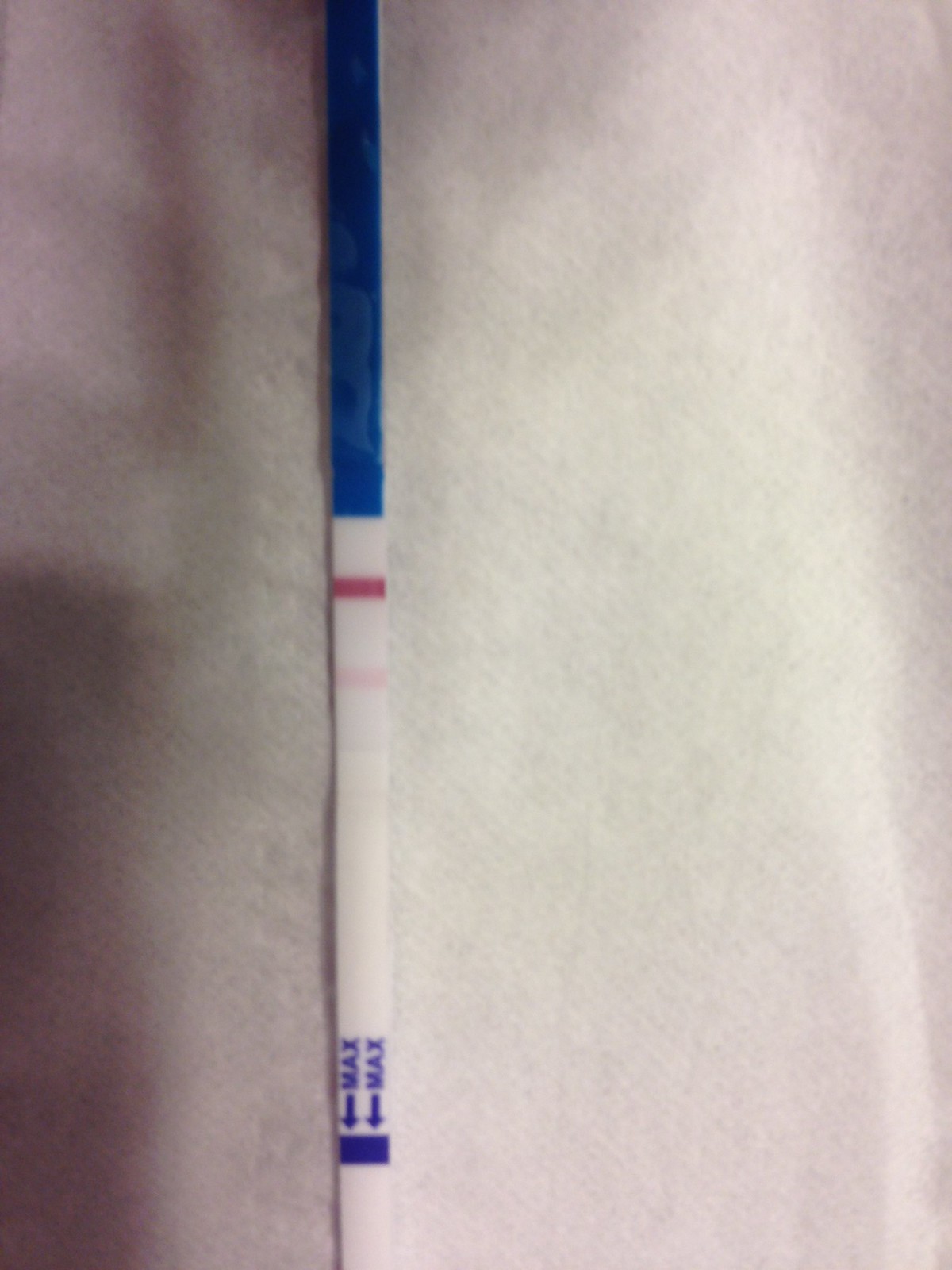An extreme close-up image displays a testing stick, prominently featuring two strips in the center. The first strip is dark red, while the adjacent strip is very faint with a hint of pink. At the bottom of the stick, blue text reads "max" twice, each word accompanied by blue arrows pointing towards a blue horizontal strip. The stick's bottom half is white, transitioning to blue towards the top, with a hint of light blue possibly due to moisture. This scene is set against a textured background that resembles a paper towel, though the close-up nature leaves its exact material ambiguous. A damp spot to the left of the stick suggests the stick was recently wet, with the paper absorbing the moisture. A subtle light area appears in the lower right corner, its origin unclear—potentially a crease or a light artifact on the paper. Additionally, a rectangular shadow is visible on the lower left side, completing the intricate and detailed composition of the image.